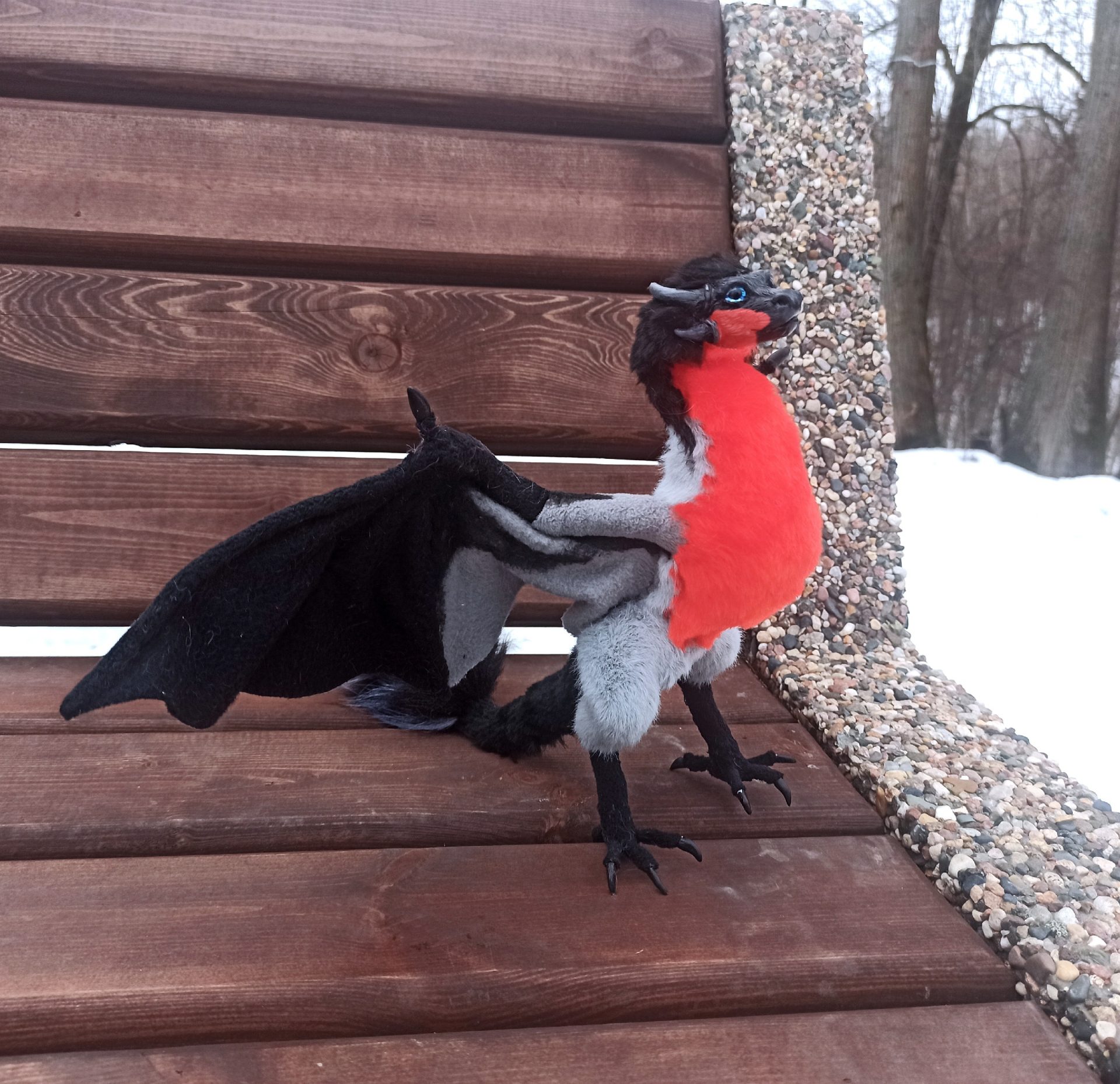This detailed photograph captures a plush, baby dragon or wyvern propped up on a wooden bench with stone supports. The scene is set outdoors in the wintertime, evidenced by the snow-covered ground and barren trees in the background. The dragon features a black head with gray horns, blue eyes, and a black snout, flanked by a black mane. Its body is a mix of plush gray with a red chest, complemented by gray legs and black claws for feet. The wings transition from gray at the base to black at the tips, and it has a black tail. Judging by its position on the bench, the toy appears to be approximately a foot tall.